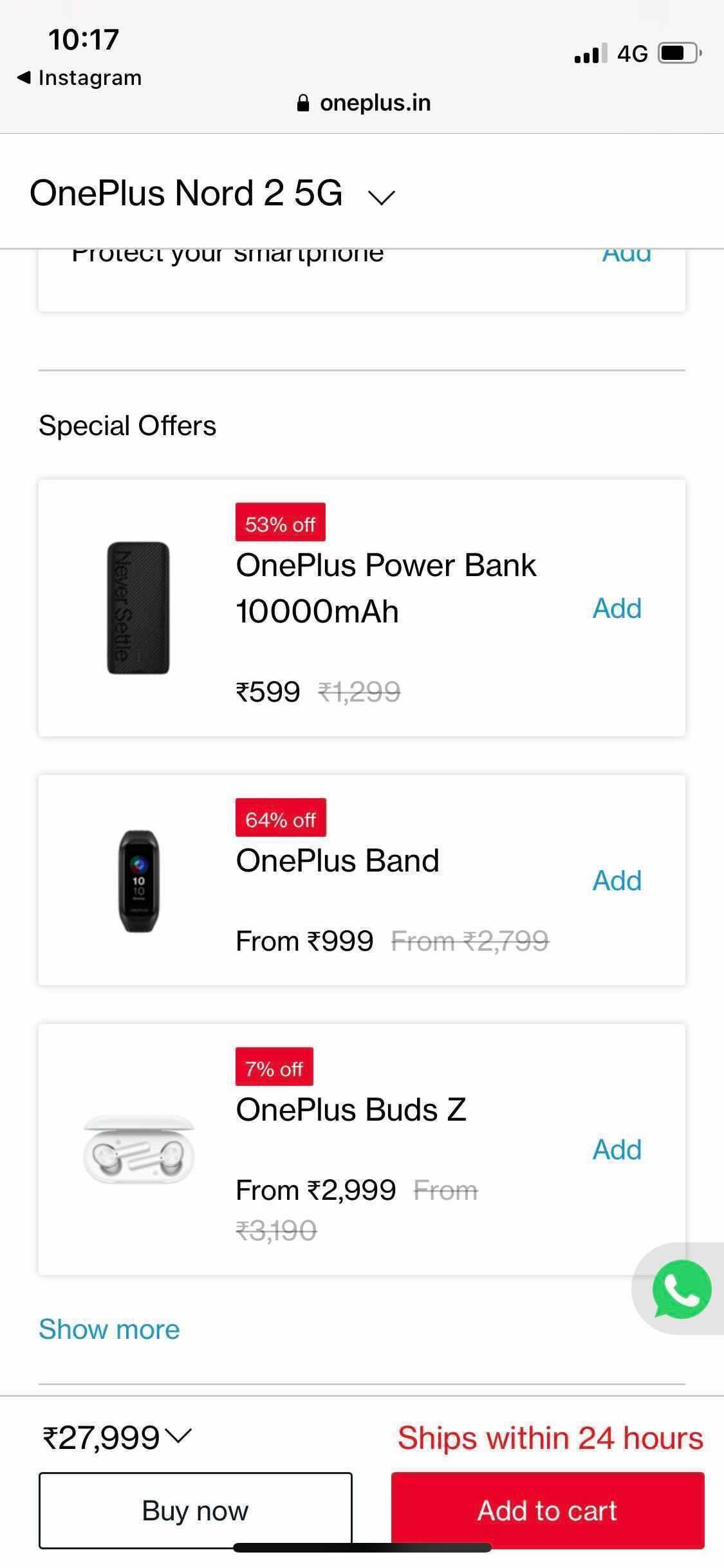The screenshot depicts a smartphone interface. In the top right-hand corner, the network coverage icon shows three out of four bars alongside the "4G" label and a battery charge icon. On the top left, the time is displayed next to the word "Instagram" and a backward arrow. The center of the grey bar features a small lock symbol followed by "OnePlus.in." Underneath it, the text "OnePlus Nord 2 5G" is shown, with a downward arrow next to it.

The main content of the screen highlights "Special Offers" with three products listed:
1. A OnePlus Power Bank with a capacity of 10,000 mAh, priced at 599 rupees.
2. A OnePlus Band, priced starting from 999 rupees.
3. OnePlus Buds Z, in-ear headphones, priced starting from 2,999 rupees.

At the bottom of the screen, two buttons are visible: "Buy Now" and "Add to Cart."